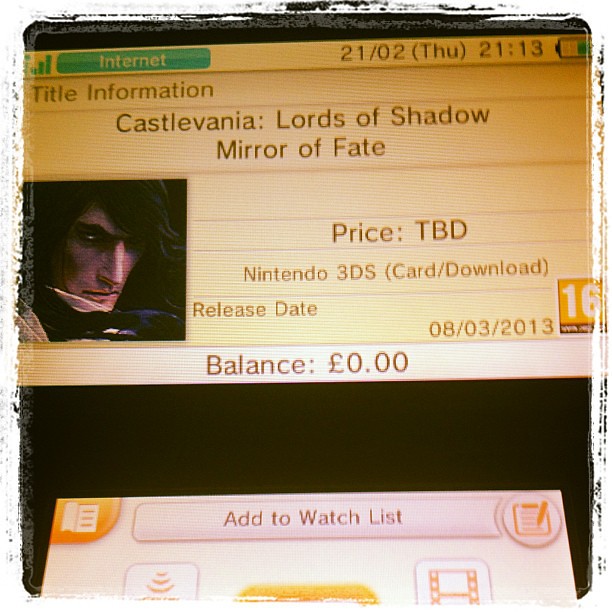The image is a close-up photograph of a Nintendo 3DS handheld video game machine's dual screens. The top screen of the device displays an online storefront page against a yellow background, showcasing the game "Castlevania: Lords of Shadow - Mirror of Fate." Key details include the title, a price labeled "TBD," platform information for the Nintendo 3DS, an option for card or download purchase, a release date of August 3, 2013, and a PEGI 16 rating. Additionally, the screen shows a balance of £0.00, a green box with "internet" and the date "21/02 Thursday 2113," and a box to add the game to a watchlist. A picture of a man with dark hair is positioned on the left side of the game title. The bottom screen features various controls that complement the top screen, helping navigate through the storefront. The device itself, which includes two LED screens and folds in on itself, is clearly identifiable as a Nintendo 3DS.